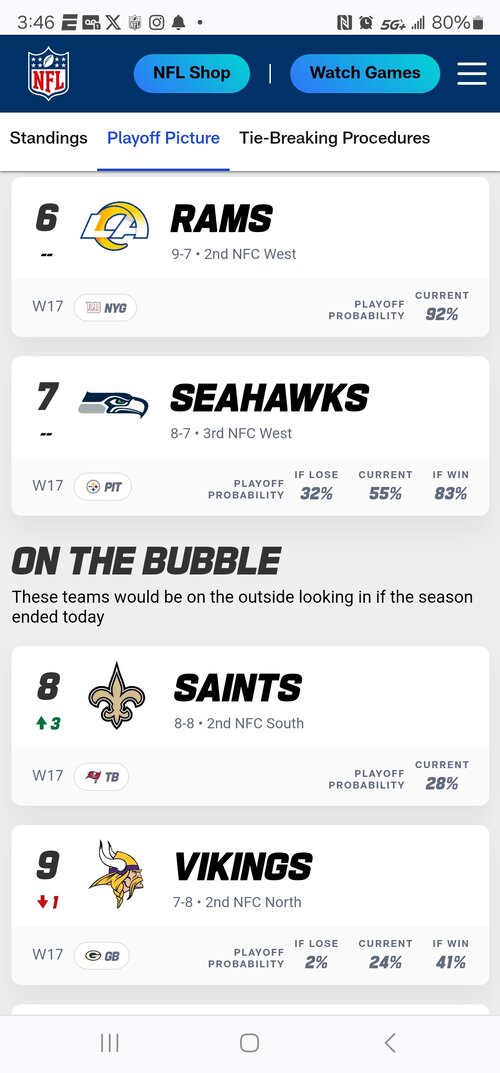The image appears to be a detailed screenshot of an NFL site viewed on a cell phone. At the top left, the familiar NFL logo in red, white, and blue is visible. Along the very top of the screen, set against a white background, is the time, marked as 3:46, flanked by additional icons: a capital letter 'E', a message symbol, an 'X', another NFL logo, an Instagram logo, and a bell. On the right side, you see an 'N', a clock icon, a '5G+' indicator, a tower strength symbol, and a battery status showing 80% charge.

Below this header, the next line features the NFL logo on the left, followed by two light blue elongated ovals marked "NFL Shop" and "Watch Games." To the far right is the menu icon represented by three horizontal white lines. Directly beneath, navigation options are listed: "Standings," "Playoff Picture," and "Tiebreaking Procedures." "Standings" and "Tiebreaking Procedures" are in black, while "Playoff Picture" is in blue and underlined, signifying the current active section.

The main content begins with a listing:
1. **6, LA Rams, 9-7, 2nd NFC West**
   - **W17, NYG**
   - **Playoff Probability Current: 92%**

2. **7, Seahawks, 8-7, 3rd NFC West**
   - **W17, Pitt**
   - **Playoff Probability If Lose: 30%, Current: 55%, If Win: 83%**

Below these entries, there's a section titled "On The Bubble," indicating teams currently outside the playoff standings:
1. **8, Saints, 8-8, 2nd NFC South**
   - **W17, TB (Tampa Bay Buccaneers)**
   - **Playoff Probability Current: 28%**
   - A small green arrow pointing up with a '3' is noted beneath the listing.

2. **9, Vikings, 7-8, 2nd NFC North**
   - A red arrow pointing down with a '1'.
   - **W17 at GB (Green Bay Packers)**
   - **Playoff Probability If Lose: 2%, Current: 24%, If Win: 41%**

The detailed probabilities suggest that the screenshot provides playoff chances likely used for betting analyses, even if betting isn't a feature on this particular site. This image captures the intricate playoff scenarios and standings for NFL teams as the season progresses.